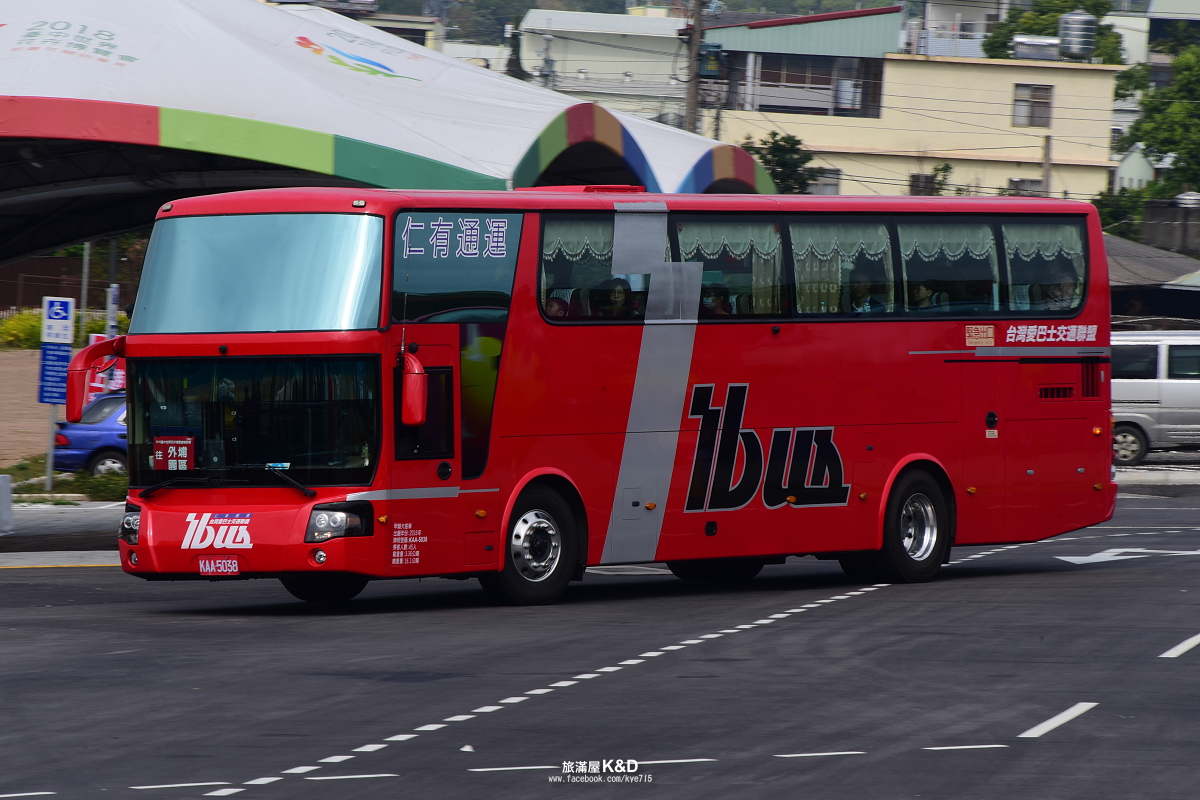The photograph captures a vibrant red double-decker bus with "I-BUS" lettering prominently displayed in the front and side. The bus is pictured from a slightly side-on angle, with the front facing the left and extending diagonally to the right. The windshield is a reflective silver, while the grille below it is black. The upper left window features Japanese characters, adding an international element to the scene. Noteworthy are the white looped curtain details visible at the top of the bus windows, adding a decorative touch, though it's uncertain if these are decals or actual valences.

The bus is positioned on a tarmac road, either parked or in motion, angled away from the lane indicated by long streaks and white dot markings down the center. Surrounding the bus in the background, one can glimpse the tops of residential buildings, a colorful striped canopy from what appears to be a market tent, with red, bright green, dark green, and yellow patterns, further adding to the lively setting. The overall atmosphere appears to be overcast, capturing a gray day in what seems to be an urban environment.